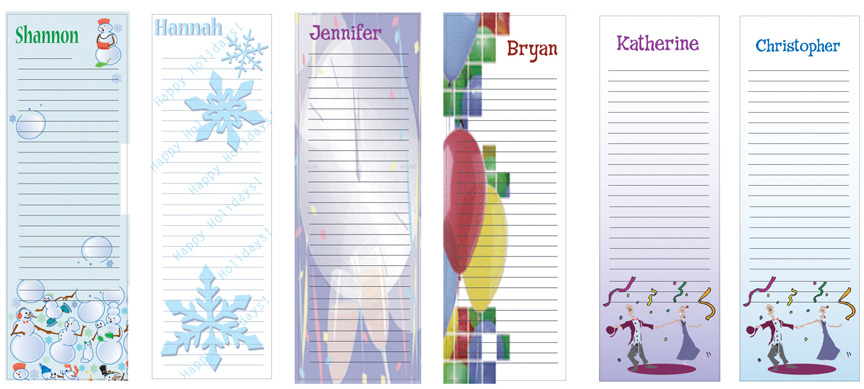This image showcases six vertically-oriented, personalized notepads, each uniquely designed for different individuals. These long, thin notepads, similar in dimension to a vertically halved A4 sheet, are designed for quick jotting and note-taking. Arranged side by side, the notepads feature names written at the top in various colors, each corresponding to specific themes:

1. Shannon's notepad is light blue with playful snowman motifs both at the top and bottom, with her name "Shannon" written in green.
2. Hannah's notepad is white with blue snowflakes and the phrase "Happy Holidays" repeated in the background, her name "Hannah" appearing in blue at the top.
3. Jennifer's notepad has a New Year's Eve theme, featuring a clock showing midnight and champagne glasses accompanied by confetti, with her name "Jennifer" displayed in purple.
4. Brian's notepad is white, featuring colorful red, blue, and yellow balloons along the left side, and his name "Brian" written in red at the top.
5. Katherine’s notepad, with her name spelled as "Katherine" in purple, shows cartoon characters of a couple dancing amidst flying party ribbons and confetti, with a purple color scheme.
6. Christopher’s notepad mirrors Katherine’s design but features his name, "Christopher," in blue atop the dancing couple graphic, with a blue theme.

Each notepad not only serves a practical function but also reflects the personal essence and celebrations pertinent to each individual.